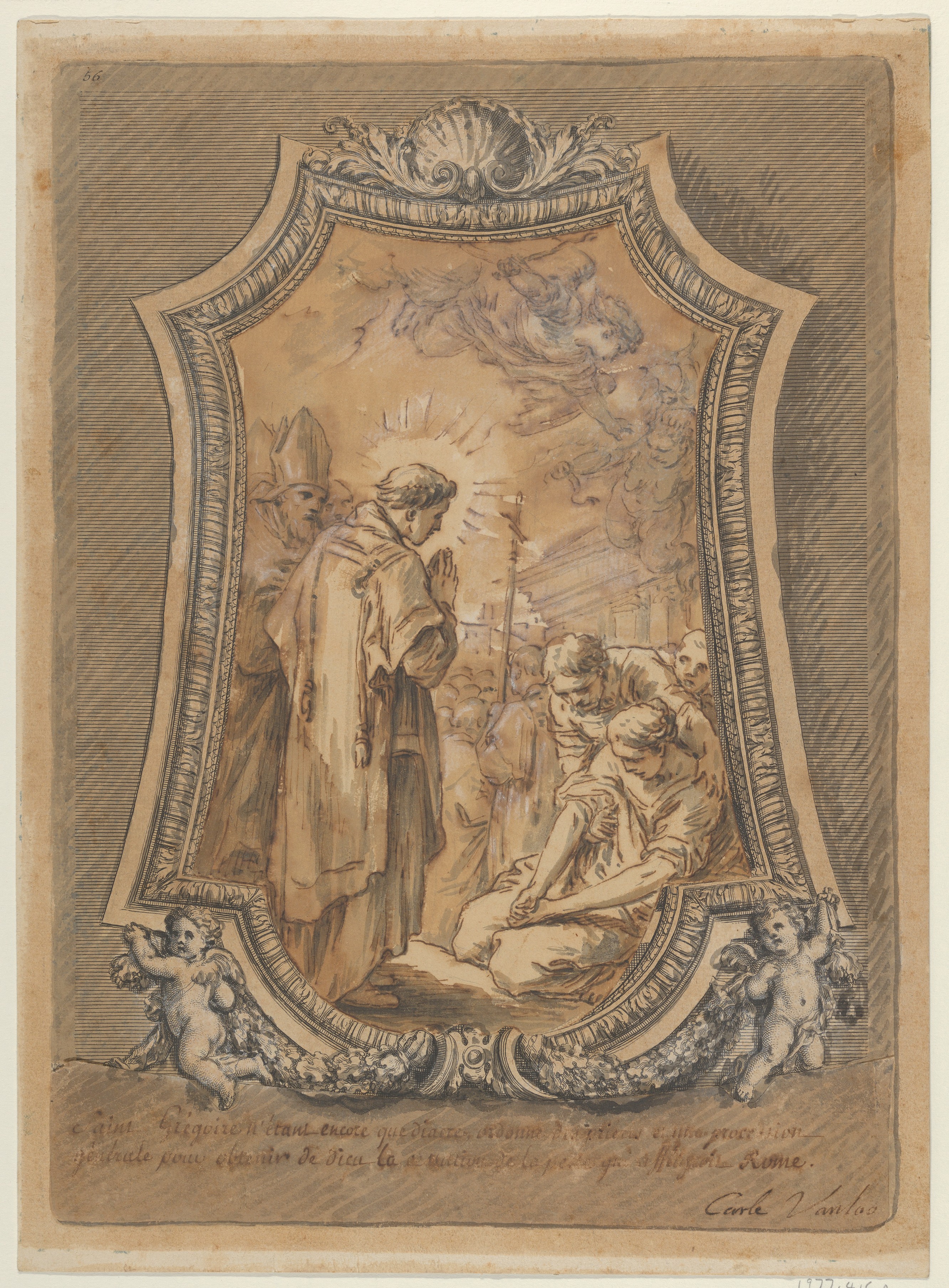The image appears to be an intricate and detailed drawing, possibly on a card, poster, or wood inset, resembling a family crest or shield. Central to the scene is a saint depicted with a halo, from which streaks of light emanate, and hands held in a prayerful position. This saint, clad in a robe that extends to his feet, is either baptizing or healing a person below him who is grasping at their legs, suggesting they are in distress. The individual being healed is supported by a hunched figure, possibly a loved one or caretaker, who has their arm around them. A bishop, recognizable by his hat, stands behind the saint, as if giving a blessing or offering support. Surrounding the central figures are additional people, including a child peering over the shoulder of the caretaker. At the bottom of the crest are two winged cupids, symbolic of divine intervention or blessing. The background of the crest features horizontal black lines, with the entire scene set against a pinkish hue, giving the image a warm, sanctified aura. There is also cursive handwriting at the bottom, possibly in a foreign language, adding to the sense of historical or religious significance.